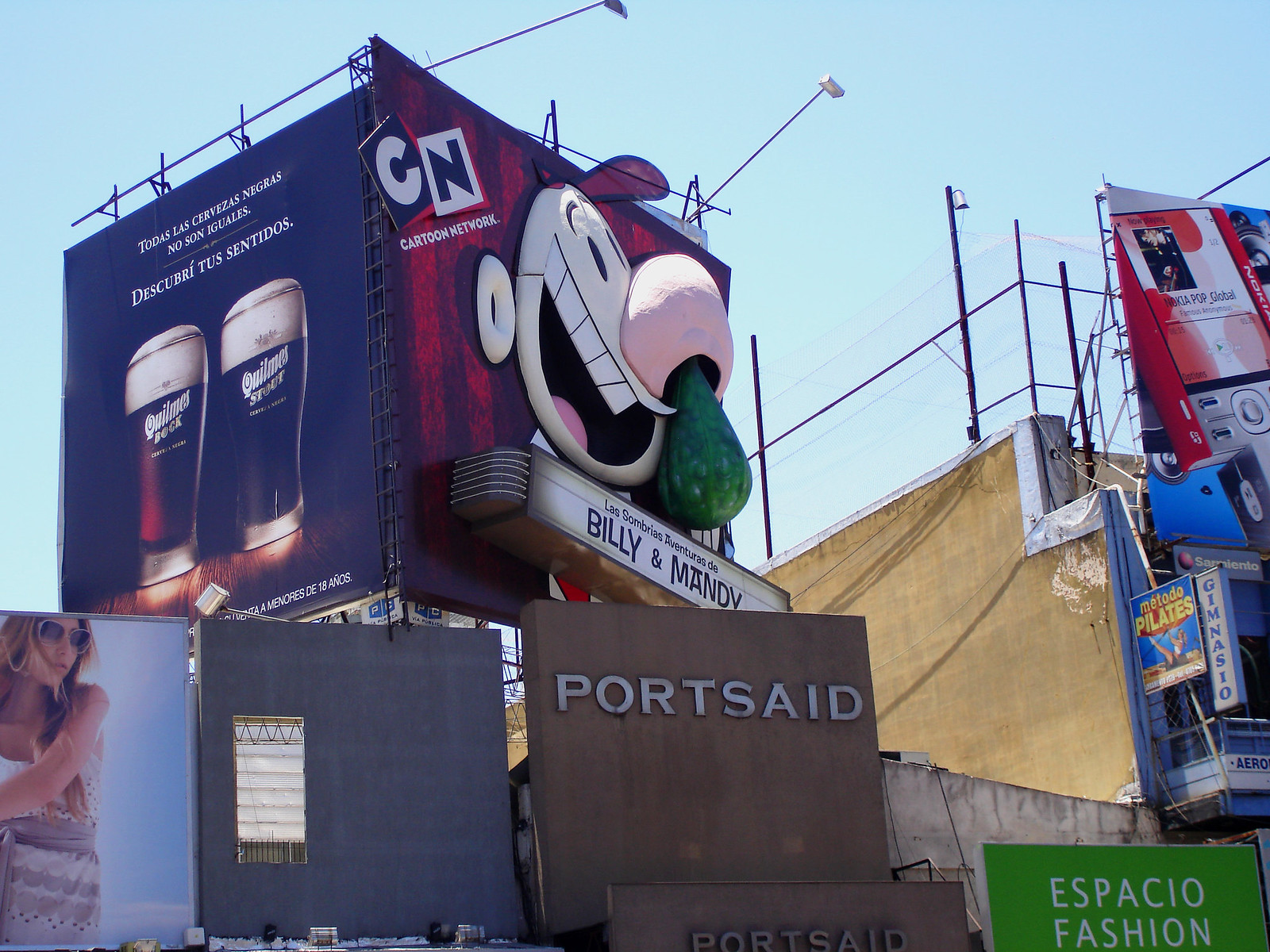This photograph captures a bustling advertisement area densely packed with various billboards atop an older building. The central billboard stands out as a Cartoon Network advertisement, showcasing a large, 3D figure of a cartoon character with a cheerful smile and a small hat, comically depicted with a green ball of mucus hanging from its nose. Above the character, there's a black and white Cartoon Network logo, and directly below it, a marquee reading "Billy and Mandy."

To the left of the Cartoon Network billboard, an advertisement for Guinness beer displays two Pilsner-style glasses filled with distinct dark and lighter brown beverages topped with foam. The sign promotes the beer with the phrase "Descubre tu Sentido," indicating a message in Spanish.

Below these prominent billboards, the area is filled with additional advertisements clinging to the buildings. There is one for "Port Said" in bold letters, another showing a female model donning sunglasses and a stylish wrap garment, and yet another reading "Espacio Fashion" set against a green background. The vibrant sky provides a pale blue backdrop to this energetic and congested urban scene.